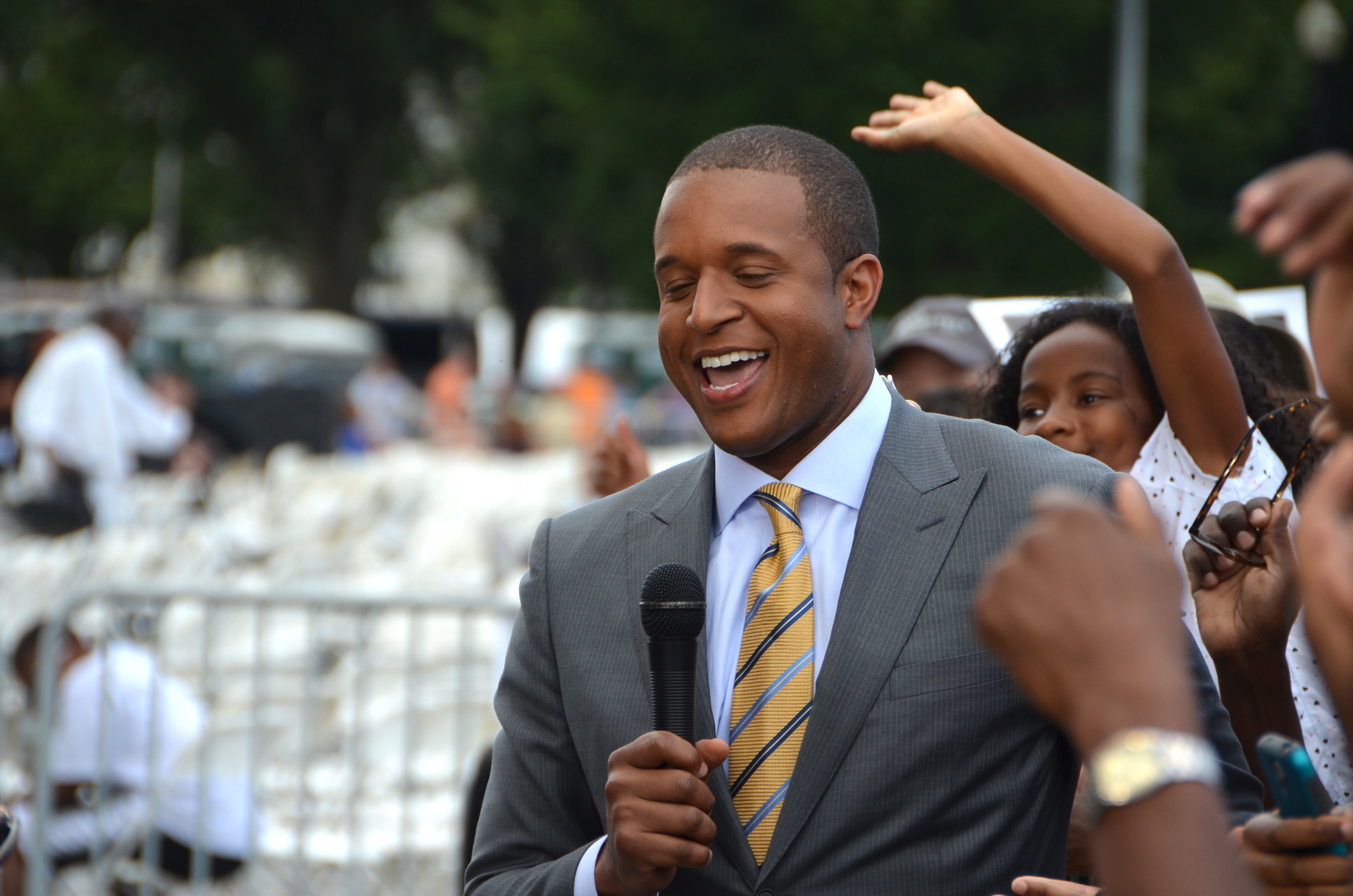The photograph features a smiling African-American man with very short hair, dressed in a gray business suit complemented by a light blue collared shirt and a yellow tie with blue stripes. He is captured from the ribcage up, holding a black microphone close to his mouth, which is wide open, revealing both his top and bottom teeth and his tongue, as if he is caught mid-speech or laugh. Situated outdoors, the background includes metal barricades and a diverse crowd of people. Among them is a little black girl, wearing a white shirt with black polka dots, who is positioned slightly behind and to the right of the man, waving her hand excitedly in the air. Further in the distance, parked cars are visible, suggesting the presence of a parking lot.